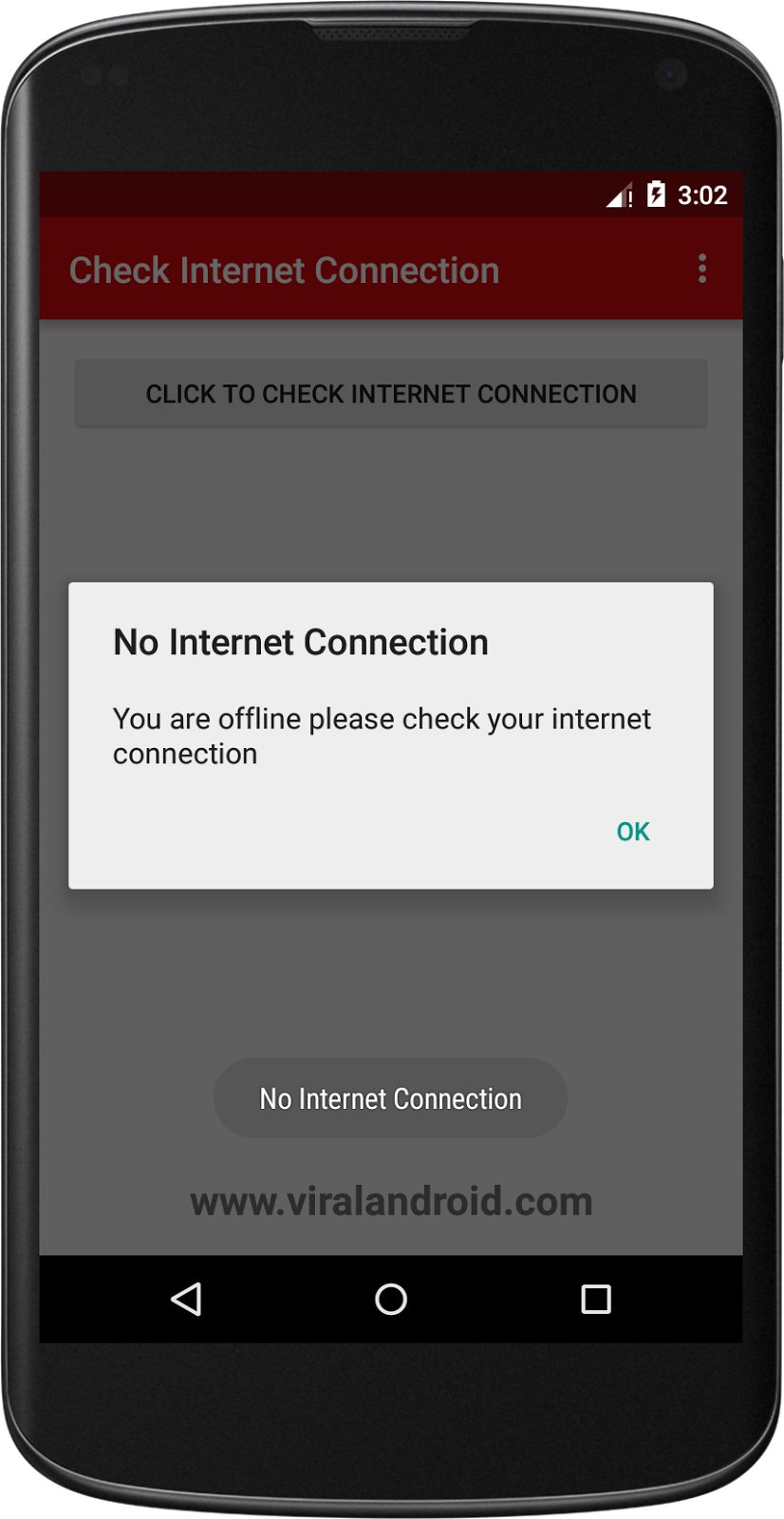The image depicts a smartphone with a black outline at the top and bottom. The screen is displaying several notifications and buttons indicating a lack of internet connection. 

At the top of the screen, the current battery percentage and time are shown. The main part of the screen features a pop-up message indicating "No internet connection" with a description advising the user that they are offline and suggesting that they check their internet connection. This message includes a prominent blue "OK" button beneath it. Lower down in smaller, gray text, the message "No internet connection" is reiterated.

Additionally, the screen features a red background banner with white text that reads, "Check internet connection," followed by three dots. Accompanying this banner is a gray button labeled "Click to check internet connection." 

At the very bottom of the screen, a gray icon with white text restates "No internet connection," and the website www.viralandroid.com is listed. Visible on the screen are three buttons: a white-back arrow, a white circular button, and a white square shape. These buttons likely serve as navigation tools or additional options, although their functionality would be limited without an internet connection.